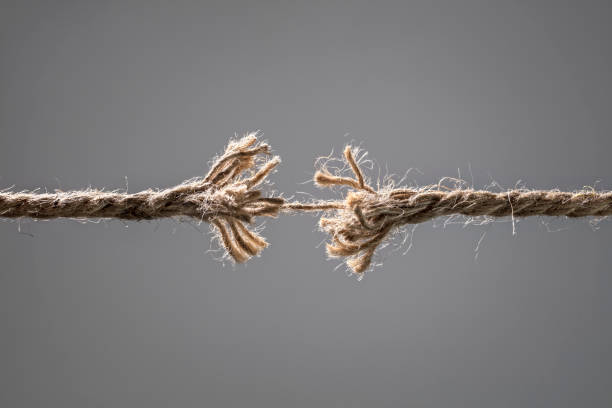The image depicts a thin, twine-like rope, woven from what appears to be twisted fiber, set against a plain, silvery gray background. This rope has been stretched to its breaking point, resulting in a frayed, almost fan-like appearance with numerous individual fibers splaying outward. At the center, a single, delicate strand remains unbroken, precariously holding the two severed ends together. The spotlight in the image seems to accentuate the fragile state of this final fiber, highlighting the intricate details of the minute strands and fuzzy, hair-like filaments that compose the rope, emphasizing its imminent snap.